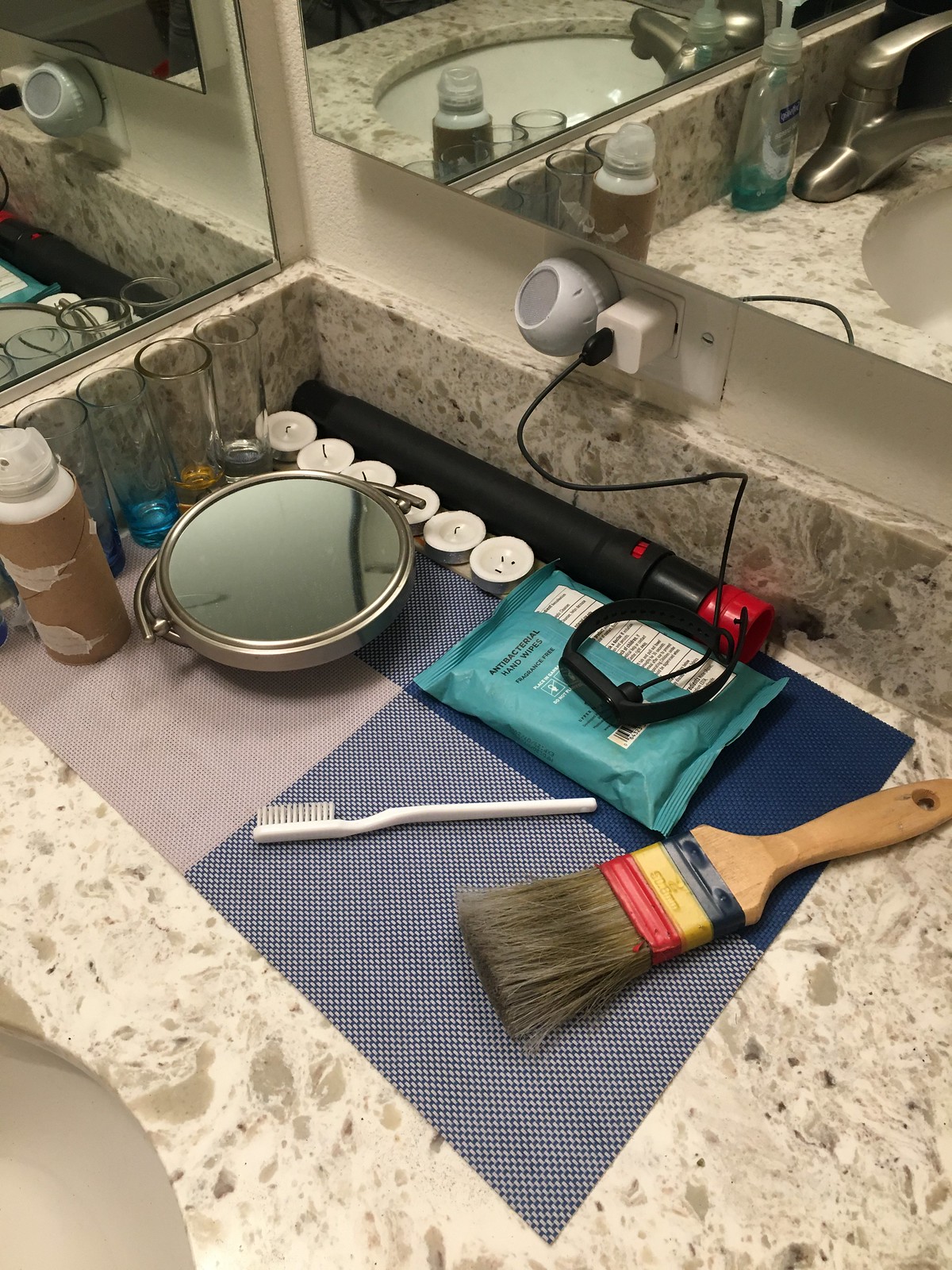This detailed photograph captures a close-up view of the corner of a bathroom sink, presented in a rectangular, portrait orientation. The image encompasses part of the adjacent walls and exhibits mirrors on both sides of the corner. 

The countertop is off-white, speckled with subtle gray and light brown spots, adding a touch of elegance. On the counter surface lies a rectangular mat, artistically divided into light purple and blue sections. The mat serves as a base for several items: 

- On the right-hand side, a paintbrush with a wooden handle adorned with dark blue, yellow, and red stripes rests.
- Just behind the paintbrush, a black and red curling iron is plugged into the wall socket, ready for use.
- To its left, a modest white toothbrush and a sleek, silver mirror are positioned together.
- A cluster of white candles is situated behind the silver mirror, adjacent to the curling iron, bringing a serene ambiance to the setup.
- A light blue package, possibly holding toiletries, is placed close by.
- Towards the left side of the countertop, a white and brown bottle stands alongside several pairs of eyeglasses, adding to the personal nature of the space.

The intricacies of the items and their arrangement on the countertop offer a glimpse into the daily routines and aesthetic preferences of the individual who inhabits this bathroom.